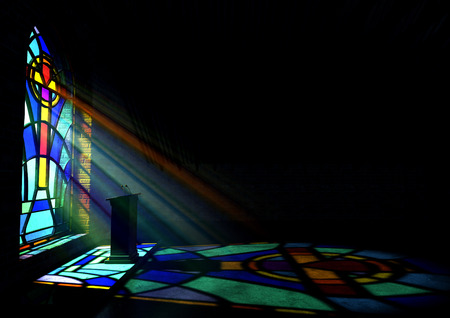The image portrays the interior of a dimly lit church, dominated by a striking stained glass window on the left side. This window, shaped as a cross, features vibrant panels of red, yellow, and purple with a background of varying shades of blue. Sunlight streams through the stained glass, casting a radiant projection onto the floor. The illuminated area displays a bright, colorful reflection mirroring the intricate design of the window, though slightly curved. The dark, black background accentuates the brilliance of the stained glass and the reflection. In the foreground, a podium stands bathed in the multicolored light. The top section of the image remains shadowed, creating a stark contrast between light and darkness.